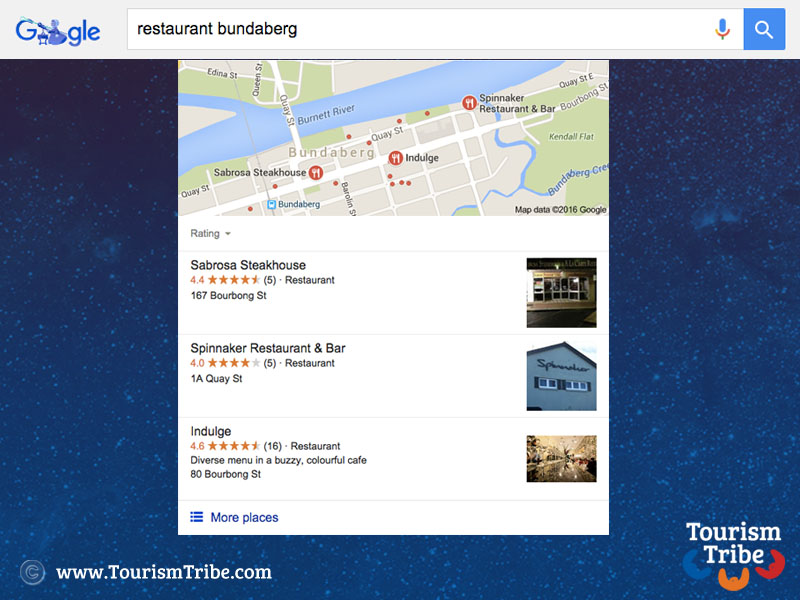In the center of this page, there is a detailed map of Banda Bek, prominently displayed against a blue background adorned with white spots resembling stars. At the bottom left corner, white text reads “www.tourismtribe.com,” and the bottom right corner features the "Tourism Tribe" logo along with blue, orange, and red colors.

At the top left, the word "Gokli" is written in blue, with the double O’s designed as illustrations of a blue-shaded old witch. A search bar is positioned at the top, containing the text "Restaurant Banda Bek." Adjacent to the search bar on the top right, there are two icons: a blue search icon and a microphone icon in blue, red, green, and yellow.

Below the search bar lies the aforementioned map. Under the map, there's a section titled "Ratings" featuring three highlighted dining options:
1. **Abroza Steakhouse** - Rated 4.4 stars by 5 people, located at 167 Babong Street.
2. **Binay Car Restaurant and Bar** - Rated 4.0 stars by 5 people, located at 1A Kwe Street.
3. **Indulge** - Rated 4.6 stars by 16 people, described as having a diverse menu in a busy, colorful café setting, situated at 80 Baobeng Street.

A text link stating “more places” is prominently displayed in blue against a white background. The map itself is color-coded with shades of blue, green, white, and grey, depicting various regions and landmarks of Banda Bek, where the restaurants are located.